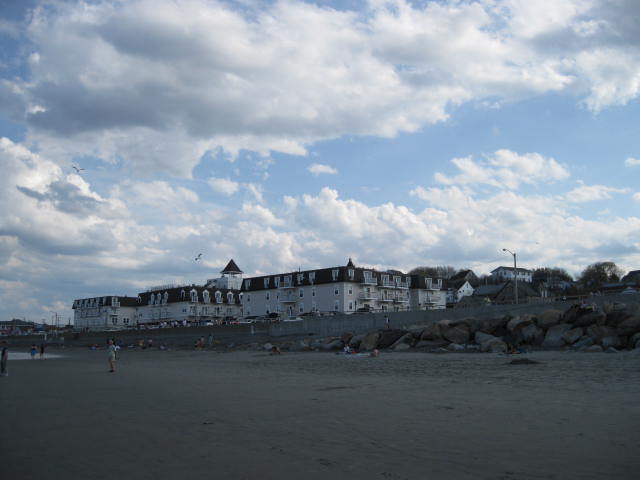The image captures a serene beach scene, possibly during early morning or late evening, as indicated by the slightly dark yet bright blue sky that dominates more than half of the frame, filled with fluffy cirrus clouds. The beach, occupying the bottom fourth of the picture, shows a mix of activities with several people strolling, standing, or resting. In the distance, a single person in a white shirt is more visibly discernible. To the right, a natural formation of piled rocks transitions into a man-made concrete wall, upon which several cars are parked and a pathway extends across the beach. Central to the composition is a large, multi-story black and white structure, possibly a mansion or hotel, with numerous windows and a distinctive red mansard roof. The building complex includes a tower featuring a conical red roof, resembling a watchtower. Along the horizon behind these main buildings, more houses and trees are visible. A light pole protrudes on the right side of the image, adding to the subtle urban elements against the backdrop of the broad, picturesque sky.